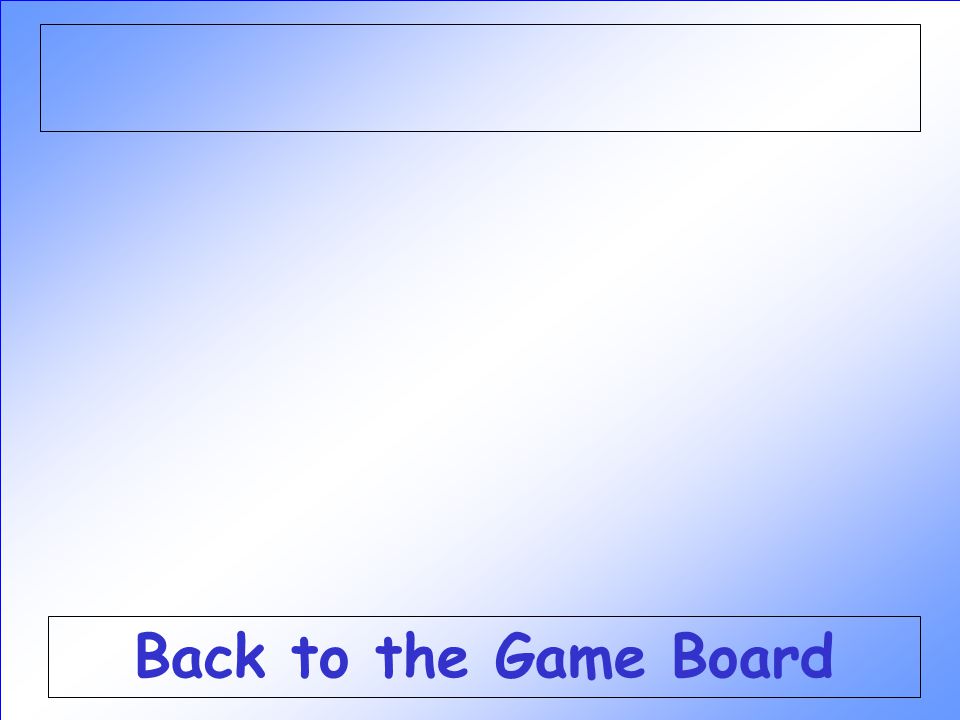The image is a rectangular illustration with a horizontal orientation, displaying a gradient background that transitions from a violet-blue at the top left corner to a lighter blue and white in the center, and back to a light blue, ending with a darker bluish-violet on the edges. The gradient creates a soft, melting effect that combines the colors smoothly. At the very top, there is a thin black-outlined rectangle, and another similar rectangle is positioned at the bottom. The bottom rectangle contains bold, hand-drawn-style text in dark blue that reads, "Back to the game board." This font appears to be written with a large marker. There are also thin black lines visible at the top and left edges of the image, adding to the detailed structure of the illustration.